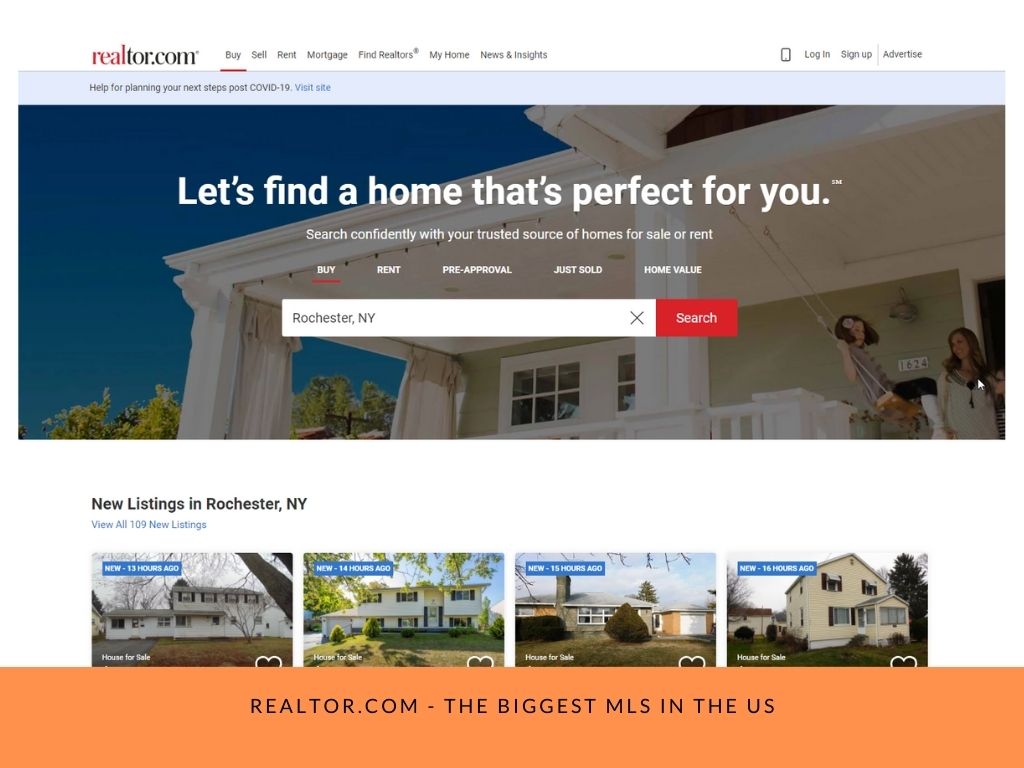The screen capture from Realtor.com features the website's interface with its logo prominently displayed in the top left corner. The top navigation menu includes options for "Buy," "Sell," "Rent," "Mortgage," "Find Realtors," "My Home," and "News and Insights." Additionally, there are buttons for "Login," "Sign Up," and "Advertise."

A banner headline provides assistance for planning the next steps in the post-COVID-19 landscape and reads, "Help for planning your next steps post COVID-19." Below it, another banner encourages users with the message, "Let's find a home that's perfect for you," set against a background image of a house. The subsequent text emphasizes Realtor.com as a trusted source for buying or renting homes, offering categories such as "Buy," "Rent," "Pre-Approval," "Just Sold," and "Home Value."

A highlighted search box with the text "Rochester, New York" pre-entered is accompanied by a red "Search" button. Underneath this section, there is an announcement of "109 new listings" in Rochester, New York, with an option to "View All." The screen shows four newly listed houses in this area.

At the bottom of the screen, an orange banner reiterates Realtor.com's stature as the "biggest MLS in the US."